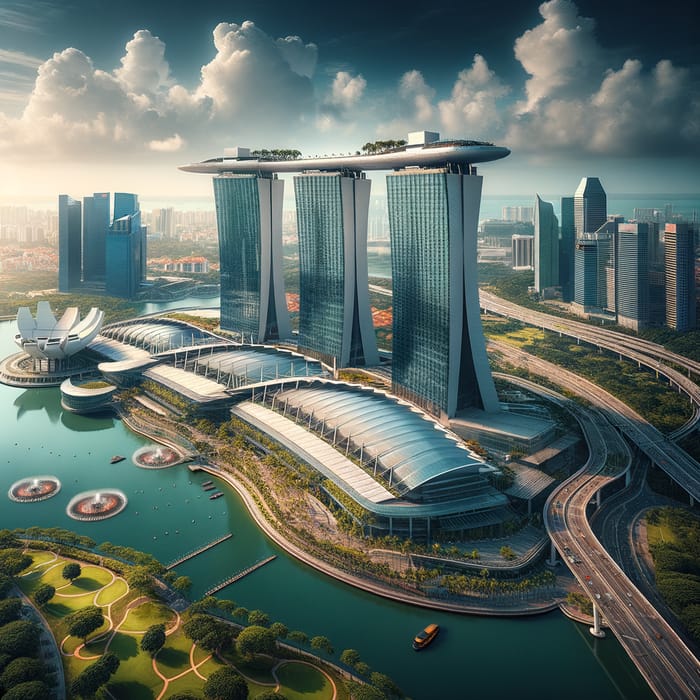The image depicts a futuristic cityscape featuring a central trio of about 50-story glass skyscrapers, interconnected at their tops by an oval-shaped, silver structure adorned with small trees. In the vicinity of these towering buildings, there are three pavilion-like structures reminiscent of the Sydney Opera House. To the left, situated in the water, is a large, flower petal-shaped building accompanied by three fountains. A bustling network of highways stretches across the right side of the image and continues into the distance where a city skyline is visible. A prominent river courses through the scene, with visible piers or docks and surrounded by lush greenery, including a golf course area. Above, a deep blue sky with fluffy gray and white clouds frames the modern vista, capturing both the innovative architectural elements and the natural surroundings.